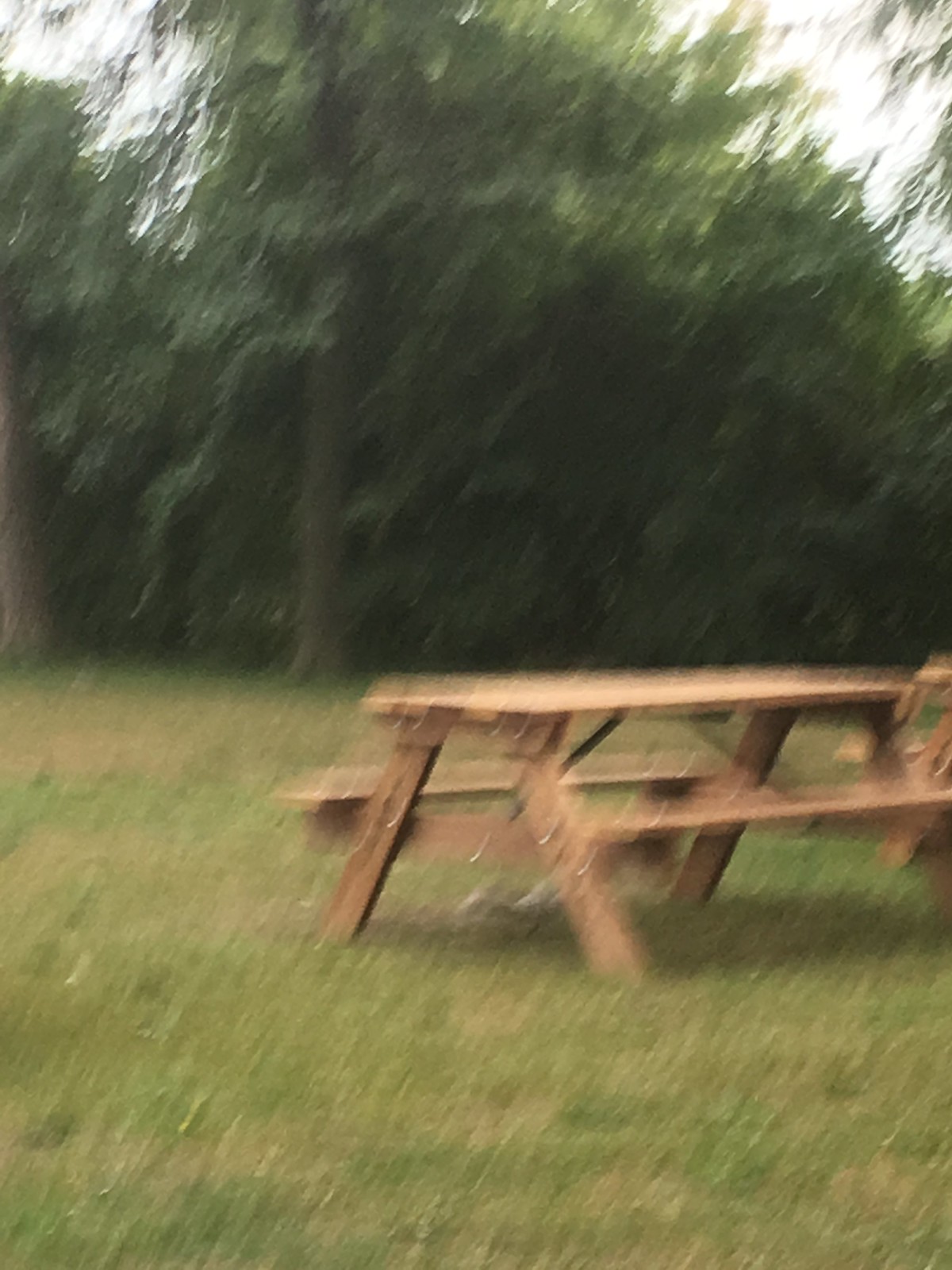In the image, there is a scene of a hazy day with dry grass covering the ground. The sky is overcast with clouds, creating a muted atmosphere. Dominating the foreground is a very tall tree with multiple visible trunks. The top of the image is filled with abundant green leaves, suggesting dense foliage. The terrain is flat and arid, indicating a lack of recent rainfall.

Positioned slightly to the right of the center is a wooden bench. The bench has a light brown seat, with legs on both the left and right sides, which are connected by a wooden board that is riveted in place. The bench seems to have an undefined object on top of it, contributing to the overall mysterious ambiance of the photograph.